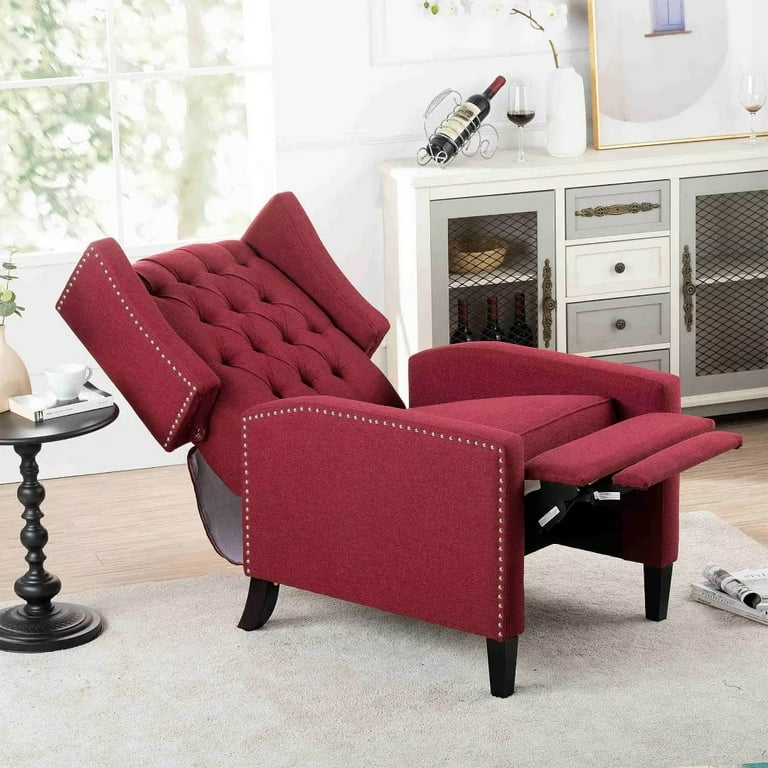In a cozy, modern living room setting, a high-end maroon fabric recliner is prominently featured. The chair, currently in its reclined position with the leg rest extended, invites relaxation with its plush, sophisticated design. Silver accents subtly adorn the headrest and armrests, enhancing its elegant appearance. Resting on a white carpet, the recliner is accompanied by a small black side table on the left, atop which sits a coffee cup on a book beside a small house plant. In the background, white shelves display bottles of red wine and glasses, contributing to the room's minimalist yet inviting atmosphere. A window with green accents is situated at the top left, adding a touch of natural light, while the overall wooden background and white furnishings complete the interior's charming design.